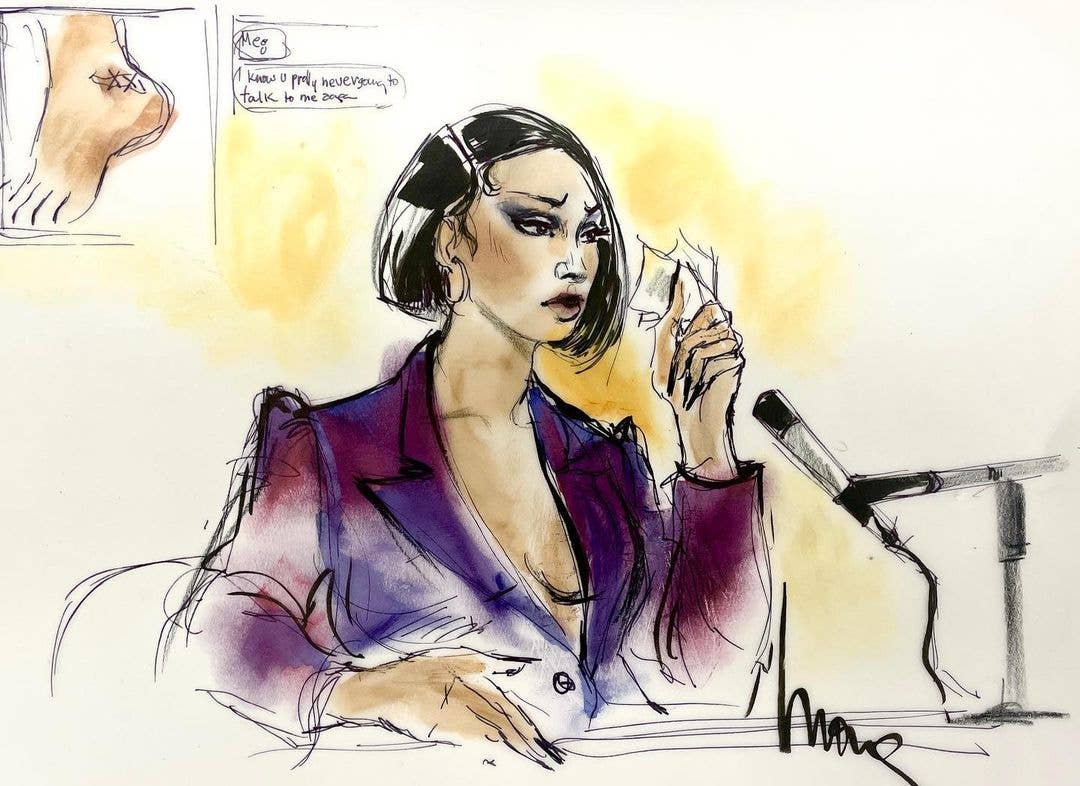The image depicts a watercolour painting or an illustration of a woman seated at the center, facing a table with a black and gray microphone in front of her. She appears worried, with a furrowed brow, possibly engaged in recording a podcast or speaking at an event. She is reading a crumpled piece of paper held in her left hand. The woman has long nails painted black and is wearing a low-cut blazer, predominantly dark purple with hints of blue, white, and pink, which is open at the front, showing some cleavage. Her skin has a tan and white complexion, and she has black and white hair. Notably, she is also adorned with hoop earrings.

In the top left corner of the painting, there is an inset depicting a brown foot with a tattoo of two stars on the ankle. Next to the foot, within a sketchy black box, there is handwritten text in black ink that reads: "Meg, I know you probably never going to talk to me again," followed by a signature. Another signature is present in the bottom right corner of the image. The background of the painting is accented with a few yellowish stains, contributing to the overall watercolor style of the piece.